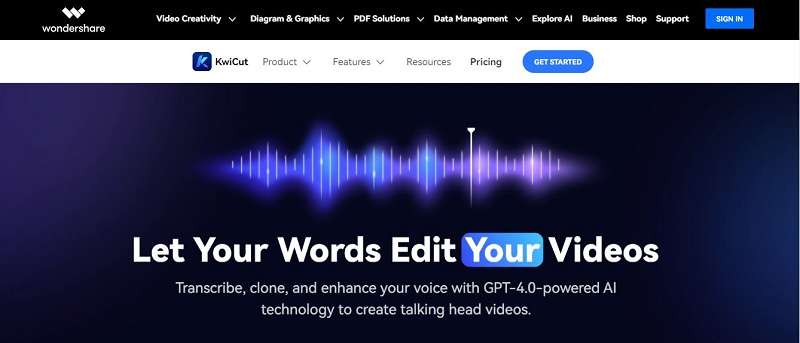This is a descriptive caption based on the provided voice caption:

---

The screenshot captures the homepage of a website branded as Wondershare, prominently displaying its W logo against a black background. The navigation bar at the top includes drop-down menus offering various categories such as Video Creativity, Diagram and Graphics, PDF Solutions, Data Management, Explore AI, Business, Shop, and Support. A blue "Sign In" button is located in the upper right corner for user access.

Below the navigation bar, on a white background, the webpage details sections for the product "Quick Cut" (stylized as "KWI CUT"), including tabs for Product Features, Resources, Pricing, and a conspicuous blue "Get Started" button.

Central to the webpage is an engaging graphic featuring a dark blue background accentuated with vertical white lines resembling a pulse diagram. Bold text reads "Let your words edit your videos," with the word "your" highlighted against a blue background. Accompanying text explains the functionality of transcribing, cloning, and enhancing your voice using ChatGPT 4.0 powered AI technology, specifically aimed at creating talking head videos. The visual and textual elements together accentuate the advanced capabilities of AI-enhanced video editing, underscoring the innovative and intriguing nature of the webpage's content.